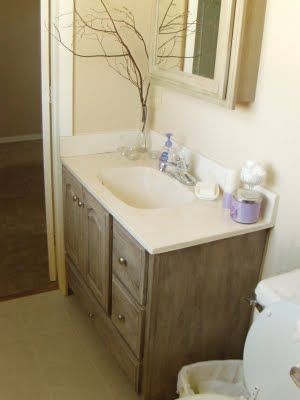In the image, we observe a bathroom corner featuring a wash hand basin perched atop an ash-colored wooden cabinet, blending tones of brown and gray. The wash basin is situated near an open door, granting a partial view into the adjacent hallway, where a dark brown carpet starkly contrasts with the light brown bathroom floor tiles. Positioned on the white countertop, alongside the wash hand basin, is a small, leafless potted plant with a skinny, brown trunk resembling a miniature tree. Additional items, including a bottle of hand soap, are also visible on the countertop, contributing to the practical yet cozy ambiance of the space.